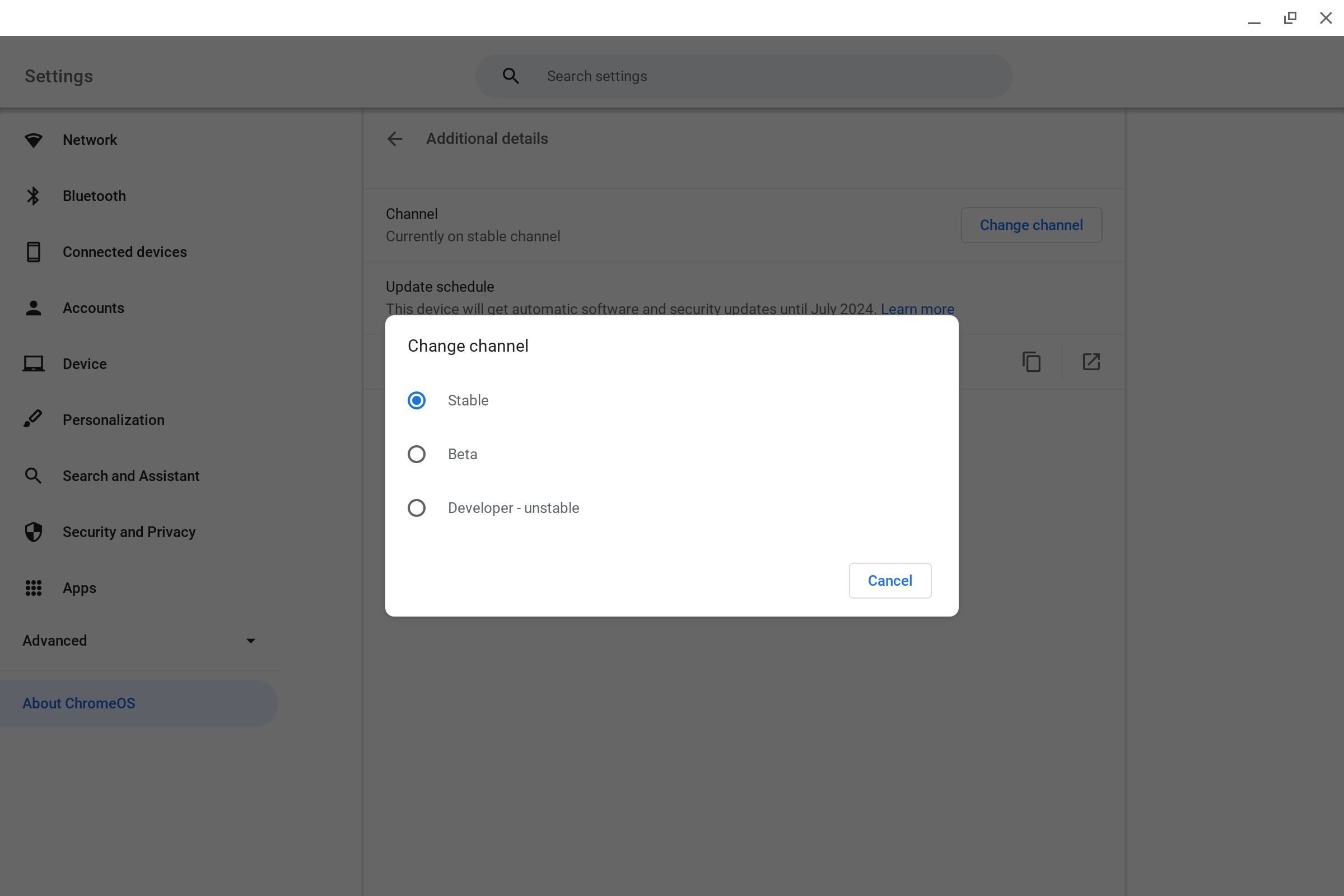The image depicts a software interface that appears to be related to network or computer management. In the background, there is a settings page with a plain white or gray backdrop featuring various options in dark text. The headings on the left side of the settings page include "Network," "Bluetooth," "Connected Devices," "Accounts," "Device," "Personalization," "Search," and "Assistant," suggesting that this is some form of network or device management software.

In the foreground, there is a prominent text box labeled "Change Channel," with options listed beneath it: "Stable," "Beta," and "Developer-Unstable." This text box indicates that the user can switch between different software release channels, ranging from stable versions to less-tested, unstable developer versions.

Behind the "Change Channel" text box, albeit partially obscured, is a notification stating, "This device will get automatic software and security updates until July 2024," along with a link to "Learn more."

Overall, the interface is minimalistic and functional, likely designed for straightforward network management or system administration tasks. The setting options and update schedule provide essential information, but the simplicity of the layout suggests a user-friendly approach.